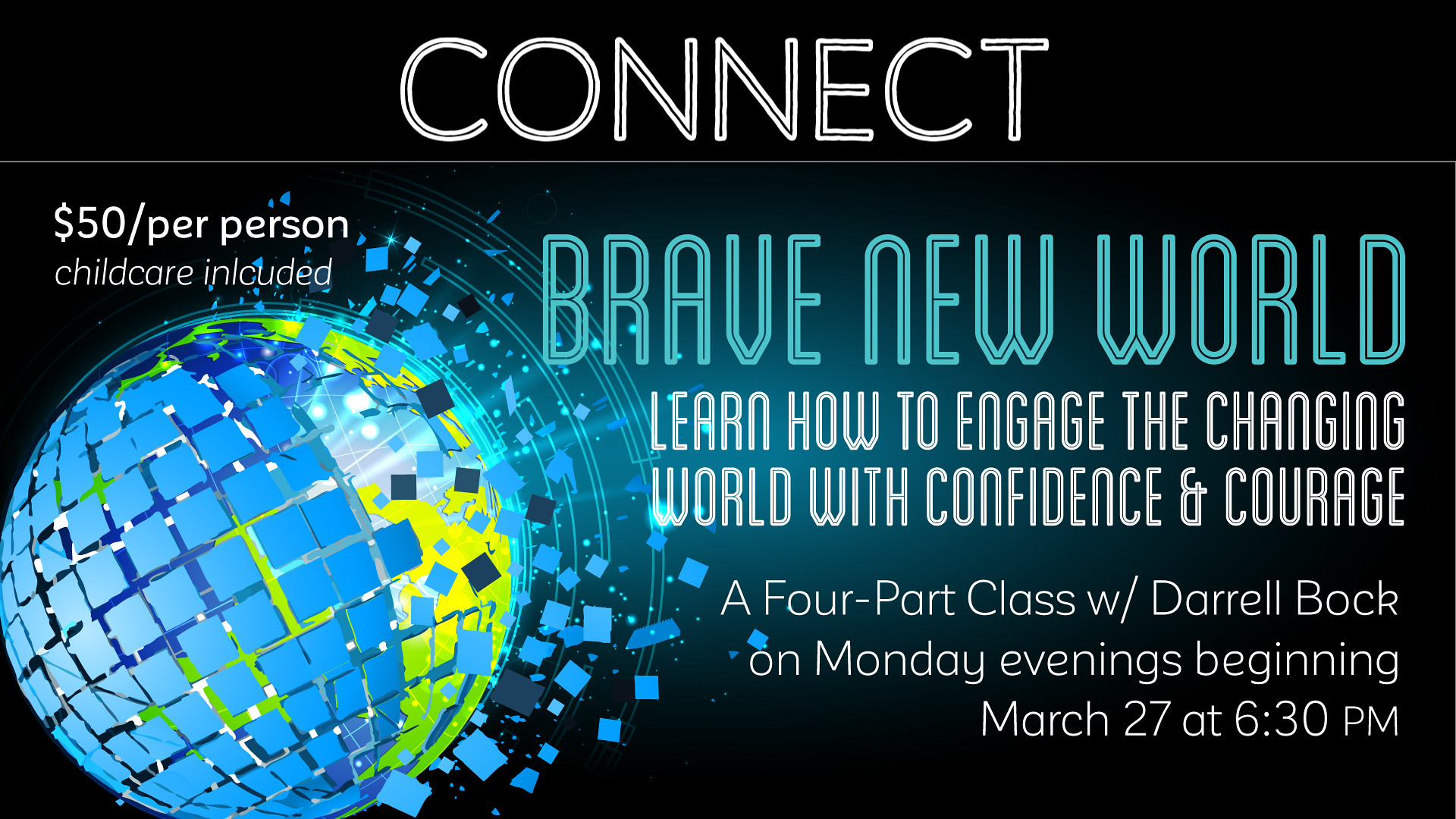The image is a digitally created advertisement set against an all-black background, prominently featuring a shattered, tile-like representation of a blue globe in the bottom left corner with yellow-green energy emanating from it. At the top, large white text reads "Connect," followed by a scrolling line underneath. To the right of the globe, over mostly the right side of the image, various details of a seminar are listed. In teal font, it announces "Brave New World," followed by smaller white text: "Learn how to engage the changing world with confidence and courage." Details about the event include: "$50 per person, child care included," and "A four-part class with Daryl Bach on Monday evenings beginning March 27th at 6:30 PM." The overall composition and style give the impression of a digital banner promoting an upcoming educational seminar. Various colors such as black, white, blue, green, yellow, light blue, and tan are noticeable throughout the image.